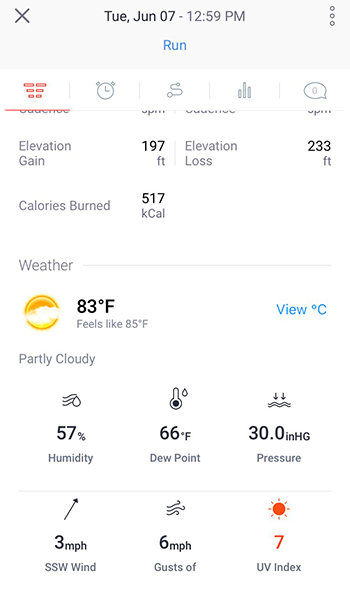Screenshot of a mobile weather application displaying detailed atmospheric conditions and additional fitness tracking data. 

At the top of the screen, a banner includes an "X" in the top left corner for closing the app, the current date, "Tuesday, June 7th," and time, "12:59 PM," followed by the word "run" in blue text, and three horizontal dots in the upper right corner indicating more options. 

The main section shows a weather summary with a small sun partially obscured by clouds, indicating partly cloudy conditions. The temperature is prominently displayed as "83°F" with a subtext in gray, "Feels like 85°F." A link labeled "View Celsius" allows users to toggle to metric units. Further details include "57% humidity, 66°F dew point, and 30.0 in HG pressure." Wind conditions are listed as blowing south-southwest at 3 mph with gusts up to 6 mph. The UV index is noted as 7, highlighted in orange for caution.

Partly cut off at the bottom of the screenshot, there appear to be sections tracking personal fitness metrics such as calories burned and elevation changes.

This informative interface conveniently combines real-time weather information with fitness tracking capabilities for day-to-day use.